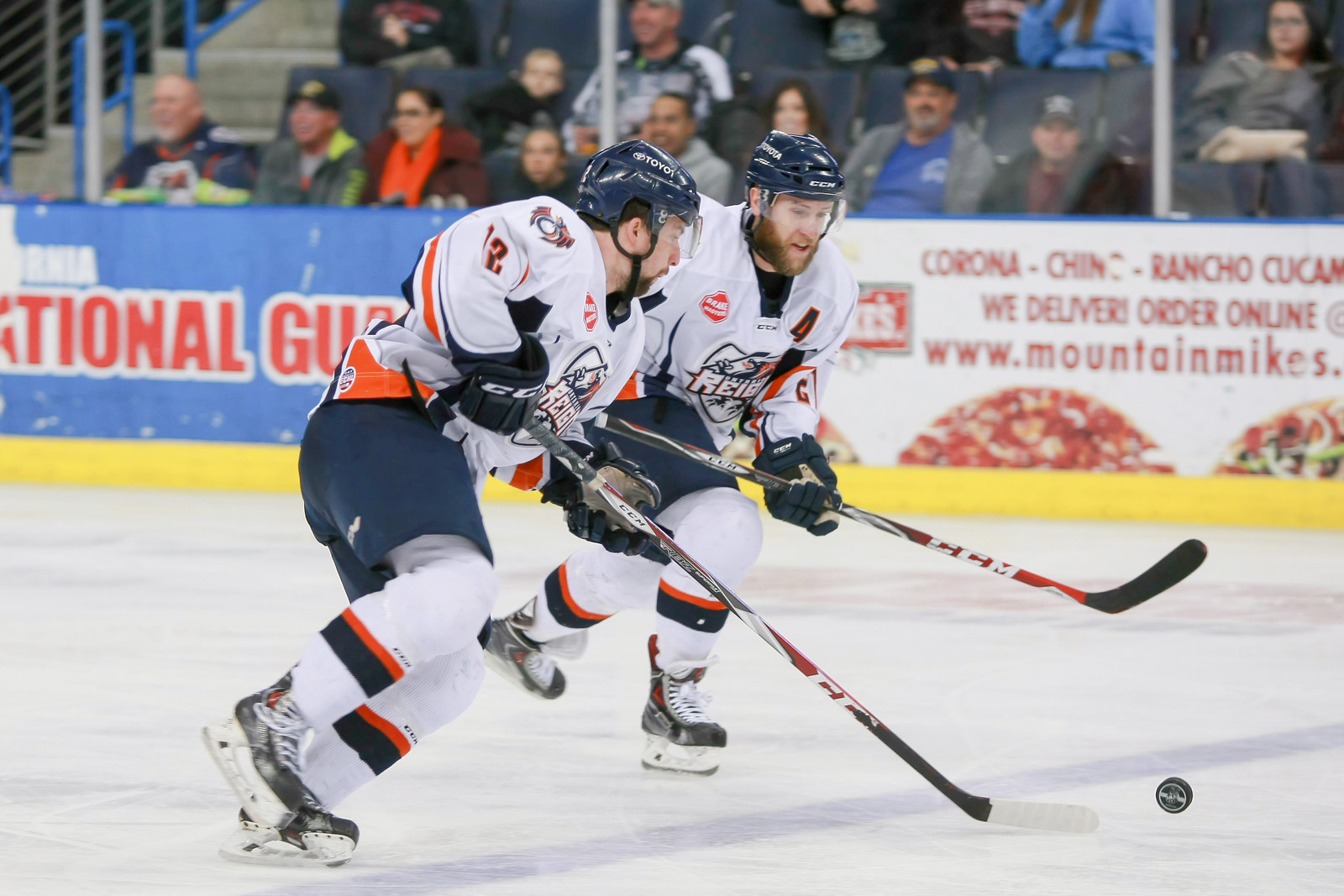In this detailed action shot of an indoor hockey game, we see two focused hockey players from the same team, distinguished by their identical uniforms — white jerseys with blue shorts, orange highlights, and blue helmets sponsored by Toyota. Both players have beards and are in the midst of racing after a puck that lies between their extended sticks, with one player's stick notably wrapped with white tape at the tip. The background features a clear view of the boards adorned with advertisements, including those for the National Guard and Mountain Mike's, with readable text like "Corona," "Chino," and "Rancho Cucamonga." Behind these boards, a slightly blurred but diverse audience watches intently; notable spectators include a man in a gray hooded sweatshirt, a woman in a bright orange scarf, and a bald man with faint green highlights on his clothing. Further in the background, blue railings line a set of stairs off to the left.